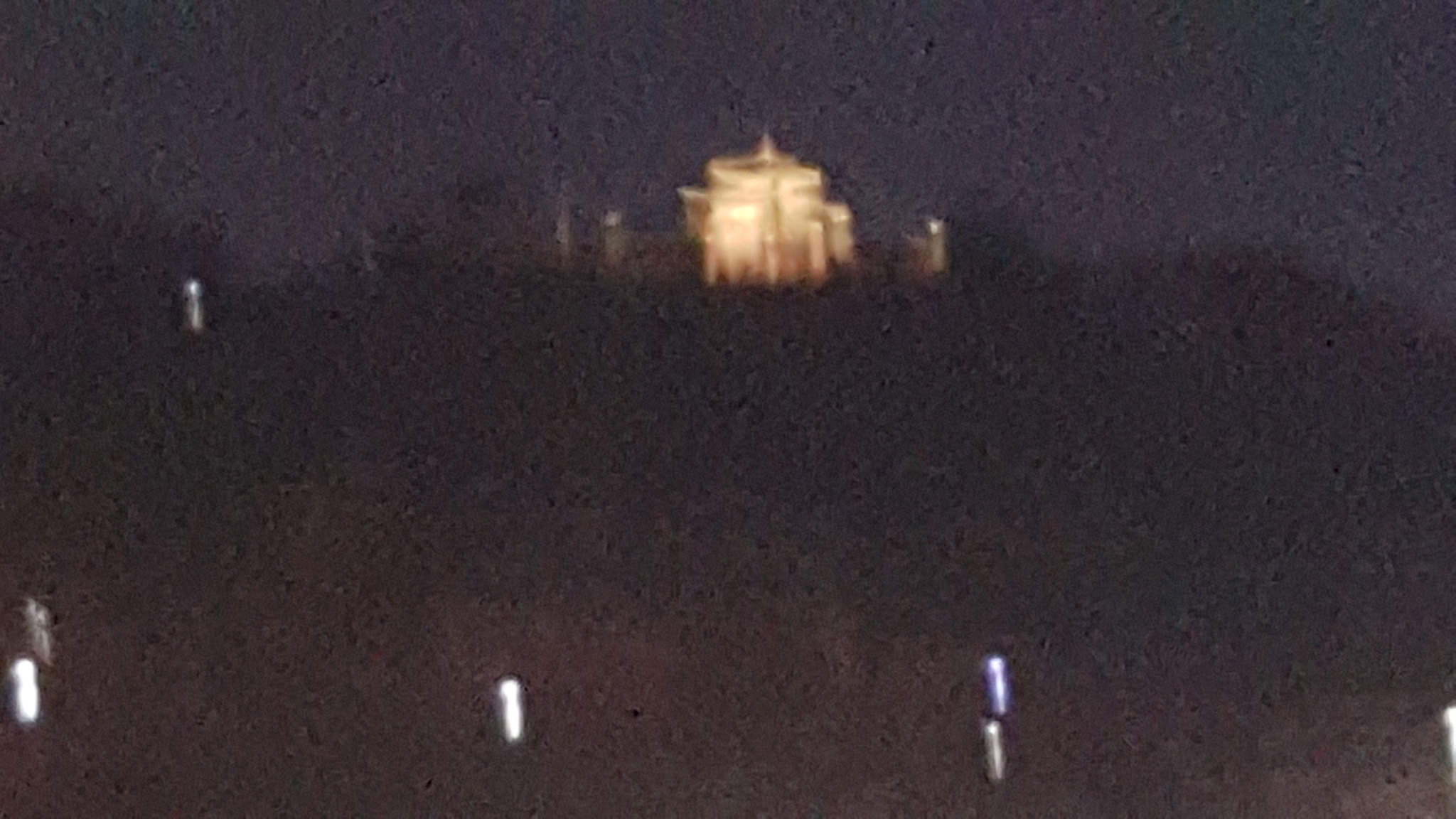The photograph appears to be a blurry, low-resolution snapshot taken at night, capturing an outdoor scene. The bottom two-thirds of the image are shrouded in shadows, likely indicating brush or landscape elements. Amidst these shadows are small white streaks, possibly light trails caused by camera motion. The focal point of the image is a glowing, Asian-style building with an ornate, circular roof that is illuminated from within. This building sits atop a hill, giving a sense of elevation. The dark sky contrasts with the dim, streaked lights in the foreground and on the building, creating a mysterious and somewhat disorienting scene. Another faint light is visible on the right side of the image, contributing to the overall murkiness and pixelation.